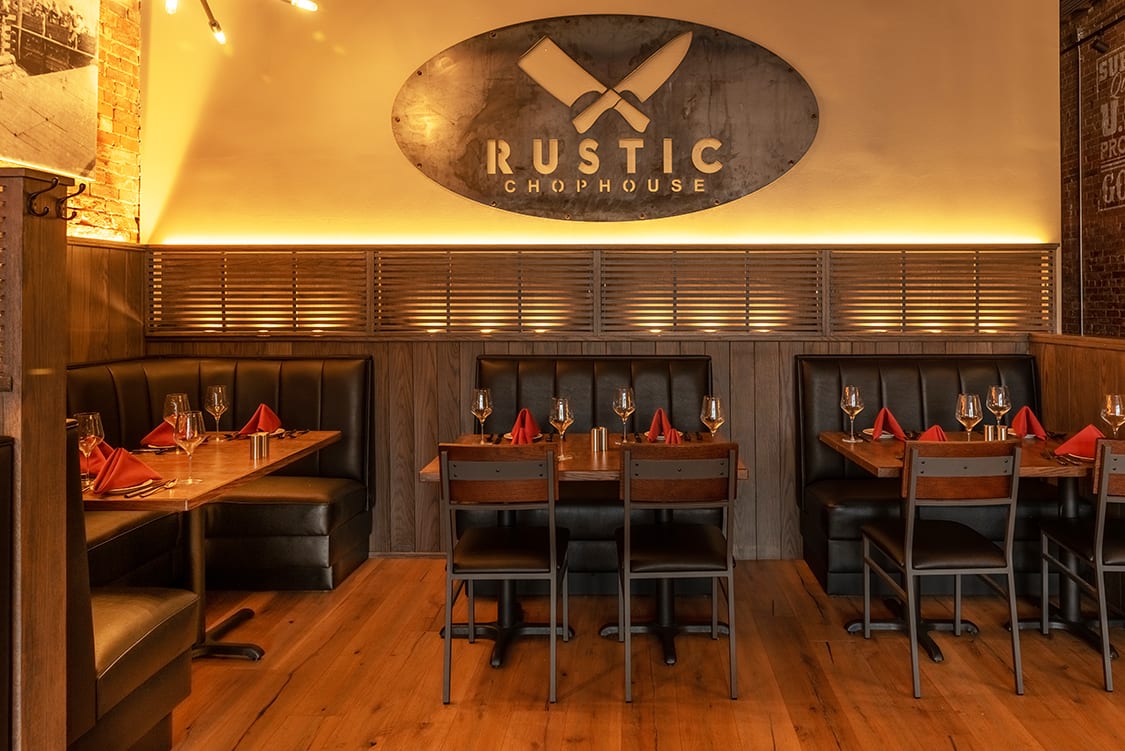The photograph captures the cozy interior of a small, hipster-style steakhouse named "Rustic Chop House." The ambiance is enhanced by dark wood paneling on the lower walls, which contrast with the illuminated, cream-colored upper walls. Yellow LED lights provide a warm glow, highlighting the wood accents and creating a welcoming atmosphere. A distinctive metal sign featuring a kitchen knife and cleaver, along with the restaurant name in stencil letters, is mounted on the wall, adding to the rustic charm.

The dining area features a mix of black leather booth seats and dark wooden tables coupled with chairs that have black frames. Each table is meticulously set with wine glasses, silverware, and red napkins folded into triangles, emphasizing the neat and clean presentation. The hardwood flooring complements the overall earthy and warm decor. There are also some vintage elements, such as a partially visible photograph on the top left wall, adding a touch of nostalgia to the modern, rustic design.